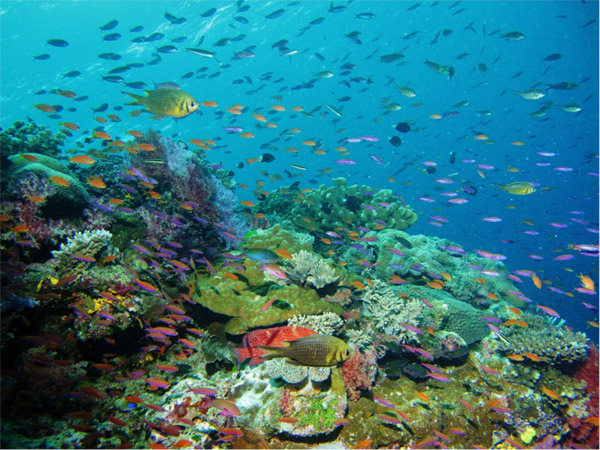This is an underwater photograph depicting a vibrant and bustling coral reef ecosystem. The crystal blue water allows sunlight to penetrate, illuminating the scene. The reef itself displays a dazzling array of greens, from dark and lime to fluorescent hues, interspersed with coral in reds, pinks, purples, and blues. Several schools of tropical fish, numbering in the hundreds, swim energetically around the reef. Among them is a striking large yellow angelfish prominently featured in the foreground. The seaweed on the ocean floor resembles confetti, adding to the dynamic and colorful impression of this underwater paradise, filled with diverse marine life and coral shapes, ranging from fern-like structures to mushroom-like formations.